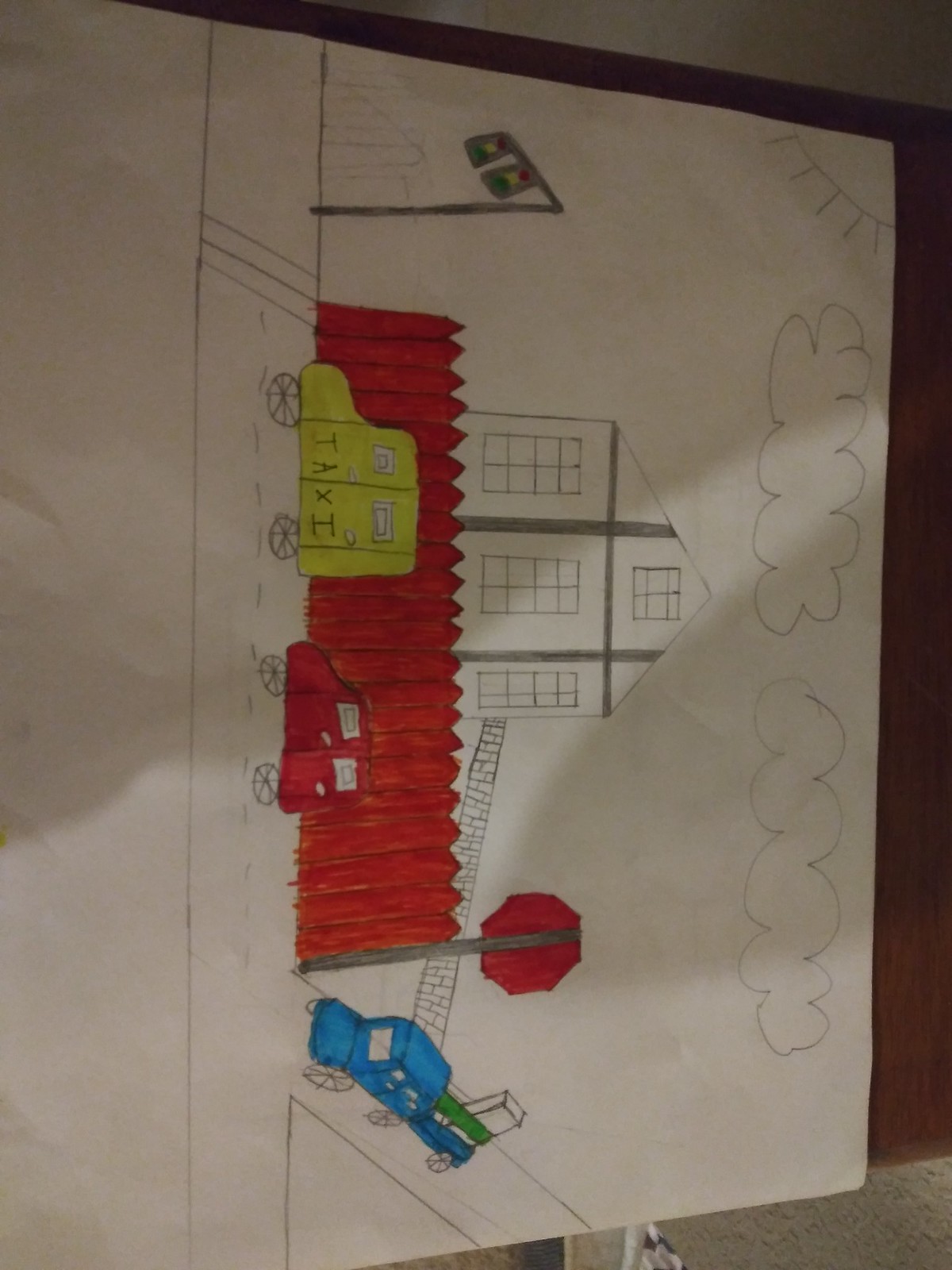A sideways photograph captures a charmingly illustrated drawing, likely the handiwork of a child. The central focus is a house with a triangular roof and a rectangular body, rendered simply in white and gray. Positioned in front is a vibrant red picket fence. To the right of the fence stands a stop sign. The scene is further animated by two whimsically drawn cars: a yellow taxi labeled "TAXI" and a small red vehicle parked in front of the fence. A blue truck is depicted coming down a road perpendicular to the house. Above, pencil-drawn clouds dot the sky, completing this quaint, youthful representation.